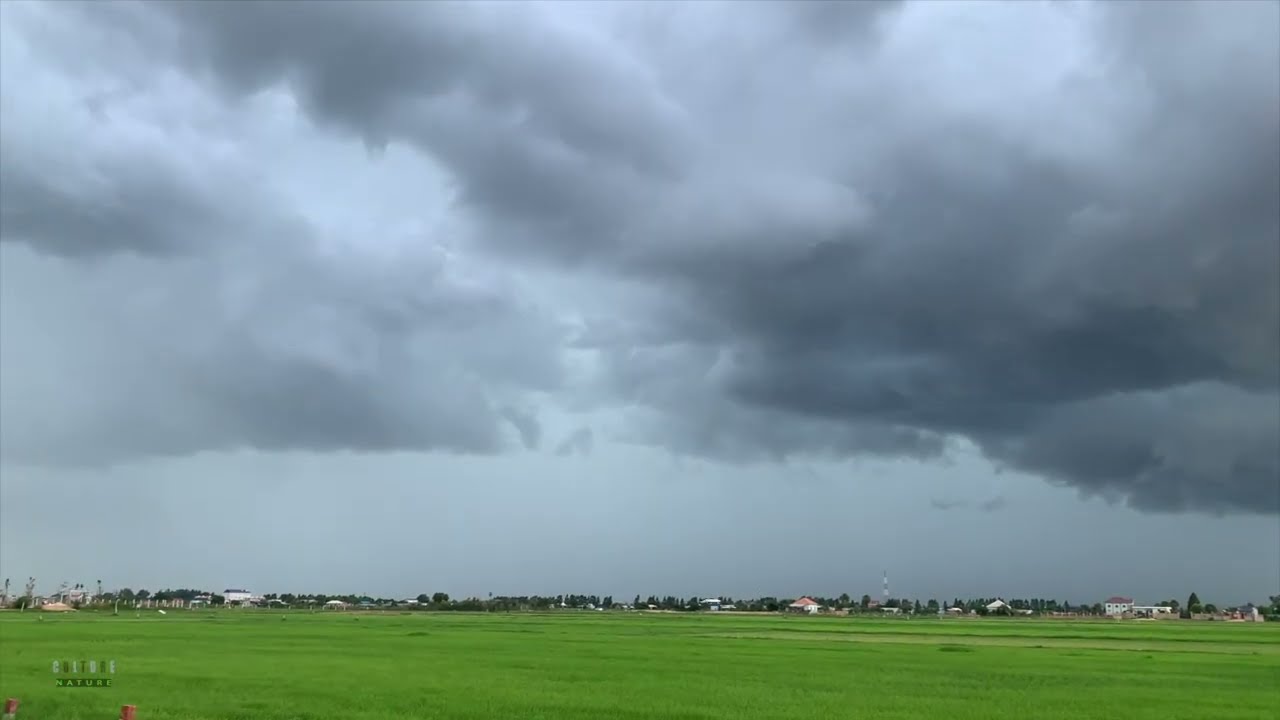The image depicts a wide open field of vibrant green grass in the foreground, transitioning into a village skyline comprised mainly of short, one to two-story buildings interspersed with trees. A prominent feature near the center is a distinctive tower with alternating red and white sections. Adjacent to this tower stands a building with a white facade and a sloped, clay-colored roof. On the left side of the horizon, a dense cluster of tall trees rises up, while on the right, another building with an arched, clay-colored roof can be seen. Dominating the sky above is a brooding, dark gray mass of clouds that grow increasingly heavy and foreboding towards the upper right corner, creating an ominous atmosphere suggestive of an impending storm. To complete the scene, there is a small logo in the bottom left corner of the image labeled "nature."